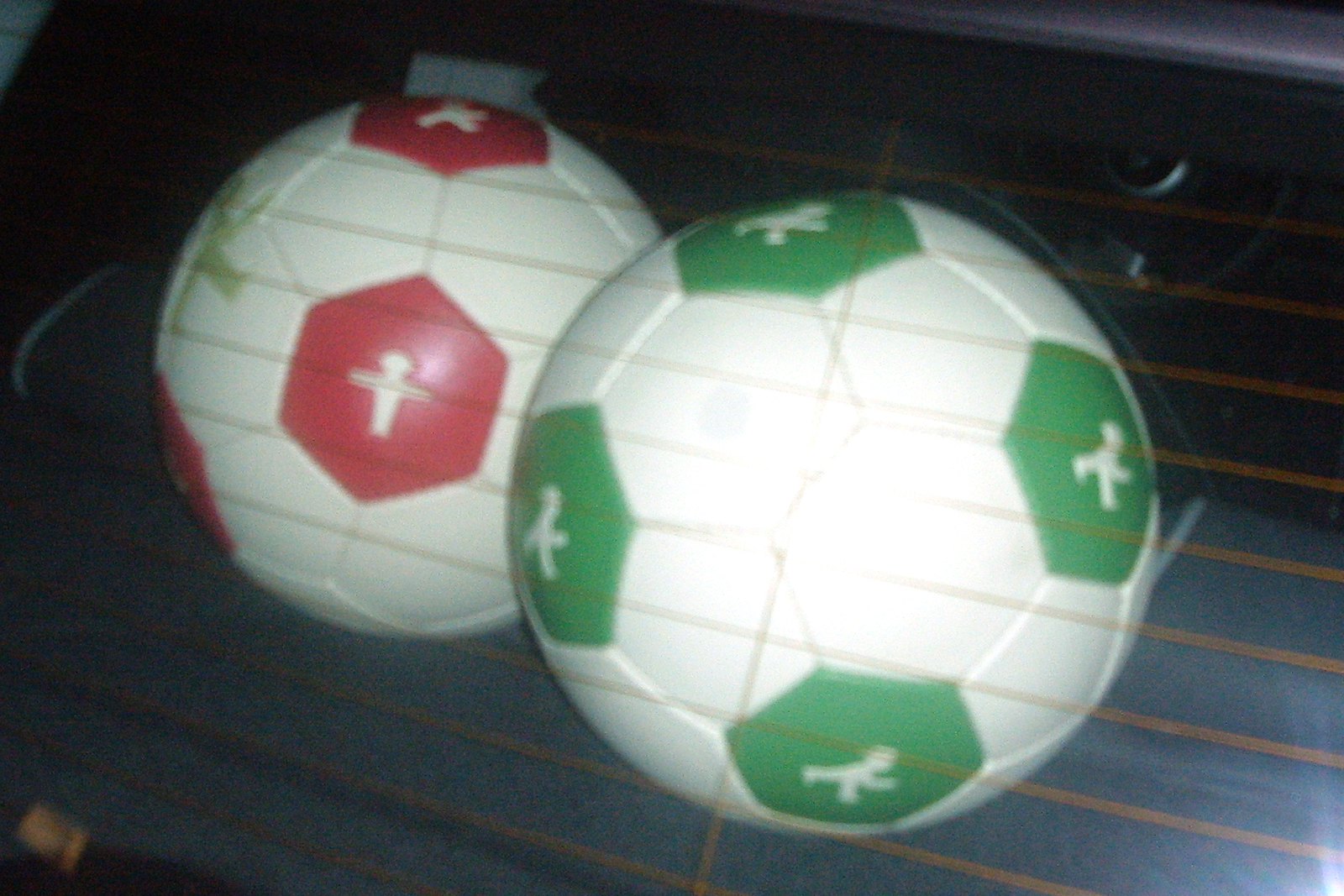This low-resolution photograph captures two soccer balls, positioned side by side, situated inside the back of a car as viewed through the rear window's heating grid. The first ball, on the left, is predominantly white with several red hexagonal patches, each decorated with an abstract figure resembling a human with arms outstretched. The second ball, to the right, also predominantly white, features green hexagonal patches depicting a more dynamic figure that appears to be in motion, possibly running. These patterns are distinctive yet abstract, with the red ball figure more static and the green ball figure more dynamic. The balls are resting on a dark surface, which could be the back ledge behind the car's rear seat. The image is overlaid by the heating lines from the rear window, appearing as yellow or brown horizontal bars, adding to the slightly obscured and dark ambiance of the picture.